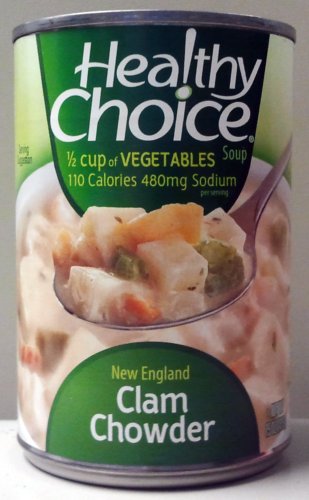This is a detailed close-up color photograph of a can of Healthy Choice New England Clam Chowder soup. The front label features the Healthy Choice logo prominently at the top against a green background. Beneath the logo, in yellow text, it states "Half a cup of vegetables," followed by nutritional information: "110 calories" and "480 milligrams of sodium per serving." The center of the can showcases a vivid image of the clam chowder in a white bowl, highlighting ingredients such as chunks of clam, pieces of carrot, celery, and peas. A silver spoon, filled with the chowder, is also visible, providing a closer look at the soup's texture and components. The bottom section of the can's label, also set against a green background, displays the product name "New England Clam Chowder" in green and white text. The can itself has silver rims at the top and bottom, framing the label.